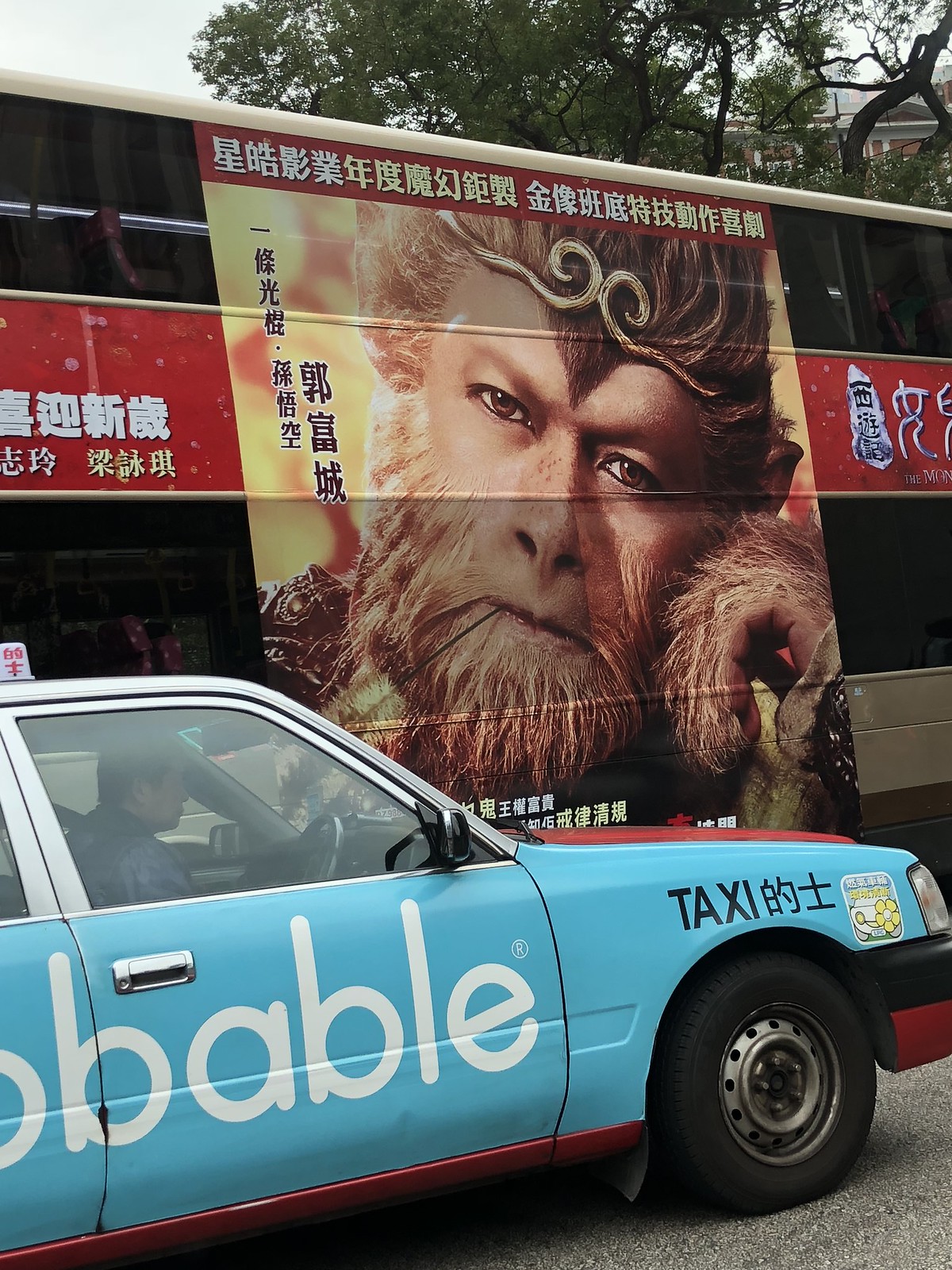The vertical rectangular image features two vehicles: a light blue taxi prominently in the foreground and a large double-decker bus situated behind it. The taxi, moving from the lower left to the upper right, prominently displays the word "TAXI" above its front right tire and features an ad on its passenger side door where the partially visible text reads "B-A-B-L-E." The bus behind the taxi is adorned with a large image of a man with a blue beard and blue, fur-covered hands, evoking the appearance of a werewolf. This striking image is set against a yellow background and is bordered with writing in oriental characters. A red stripe runs between the bus's first and second levels, right beside the vivid image of the man. In the far background, behind the bus, there are trees, completing the urban yet slightly surreal scene.